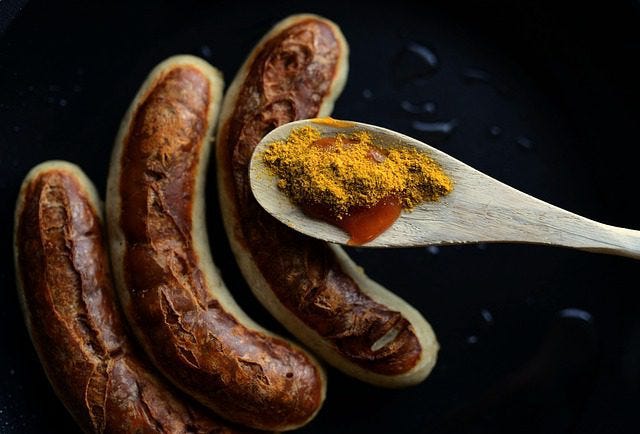This top-view photograph captures a culinary scene with vivid details. On the left side of the image, three well-cooked, reddish-brown sausages, reminiscent of hot dogs or wieners, are arranged neatly in a black frying pan. These sausages have a distinctive C-shape, curving up and to the right, and their browned tops contrast with the cream-colored sides, suggesting they are thoroughly fried. The glossy black background of the pan is slightly dotted with water droplets and oil, adding a touch of realism to the scene. Crossing the right side of the image into the center is a gray wooden spoon. This spoon holds a red liquid, likely honey or syrup, with a fine, yellow powder sprinkled on top, possibly mustard or turmeric, presenting a mouth-watering blend of colors and textures. The spoon and sausages together create a visually appealing and detailed snapshot of culinary artistry.